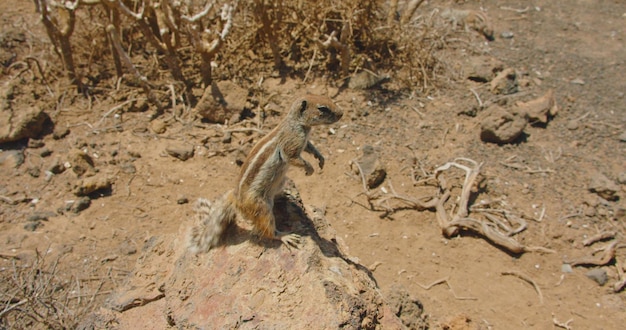This rectangular photograph captures a slender squirrel, possibly a chipmunk, standing upright on its hind legs on a small, soil-covered rock in an outdoor setting resembling a dry desert environment. The squirrel, with its reddish-brown, gray, and white-striped fur, is positioned centrally, facing towards the right, allowing us to see its side profile and bushy tail. The ground, primarily brown due to the dirt and soil, is scattered with additional rocks, smothered stones, and remnants of dried vegetation, including a dead bush nearby. The overall scene conveys the arid, rustic habitat of this small creature, enhancing the naturalistic context of the image.